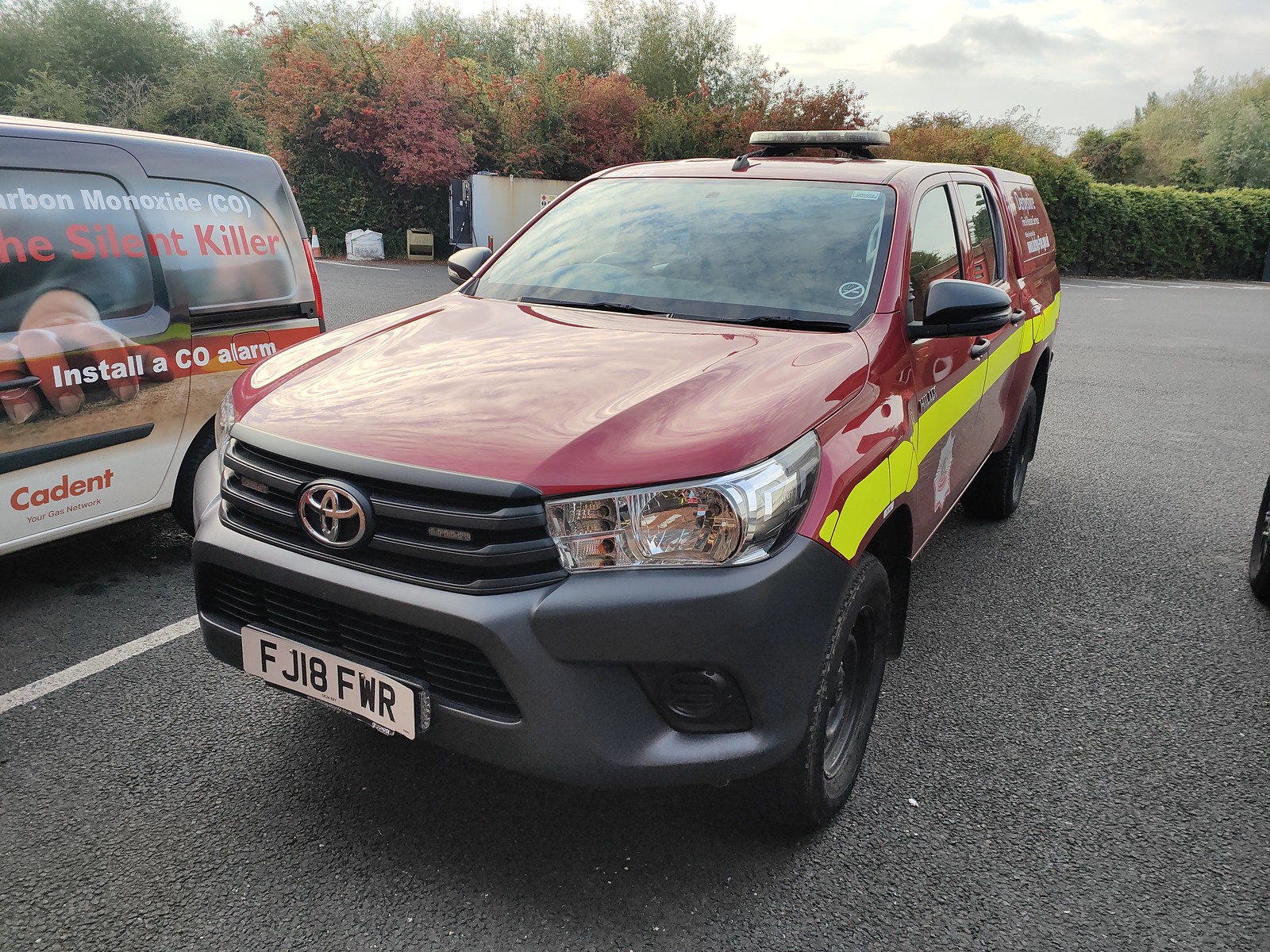This detailed image depicts a red Toyota SUV, likely a Tacoma, viewed from the front in a parking lot. Distinctively, a reflective neon yellow stripe runs along the entire length of the driver's side from front to back. The vehicle boasts a sturdy black bumper with a matte finish and a white rectangular license plate with black lettering that reads FJ18FWR. Atop the SUV, a light bar is mounted behind an antenna, reinforcing its role as a possible service or rescue vehicle. The SUV features black tires with matching black rims and has white lettering on its rear. Parked to the left is a van adorned with multiple brandings, including a graphic of a hand and text that warns, "Carbon monoxide, the silent killer." The setting appears to be a cool, overcast day, with trees, shrubs, and bushes visible in the background.